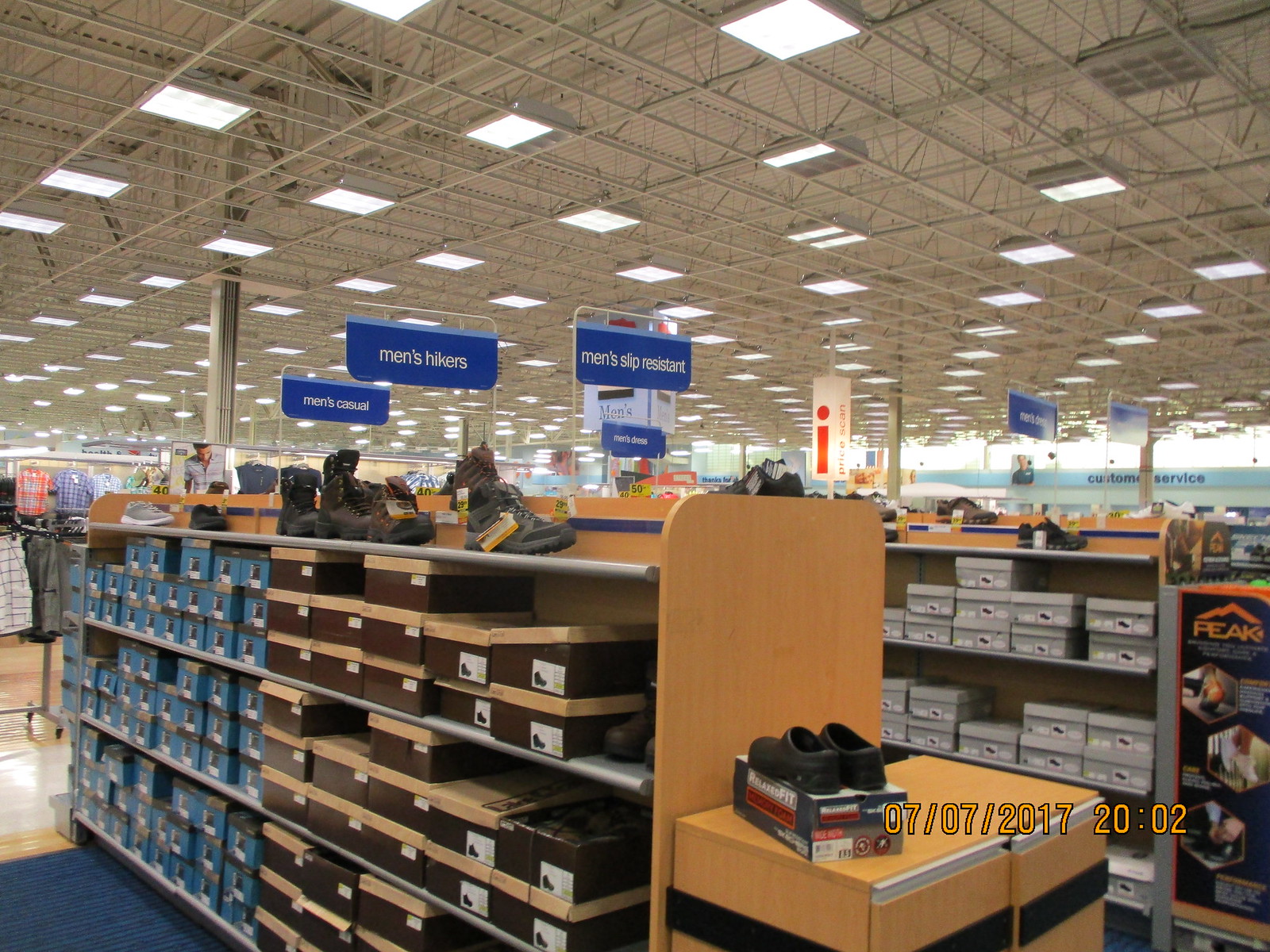The image depicts a bustling shoe store, specifically the shoe department. In the bottom left corner, a blue rug is visible, adjacent to a rack of clothing items, all set against a brown floor. To the right of this rug stands the first shelving unit filled with boxed shoes. Displayed on the top row of this unit are various shoes, while the boxes below are organized into three horizontal rows, with brown boxes on the right and blue boxes on the left. The shelving unit itself features a light brown exterior. On top of the gray box at the right edge of this unit, a pair of black shoes is prominently displayed. Further to the right, a yellow date stamp reads "07-07-2017-2002." The scene extends to show more shoes and miscellaneous items for sale, with blue signs hanging from the ceiling. The ceiling is gray and dotted with square beams of light at regular intervals, providing ample illumination throughout the store.